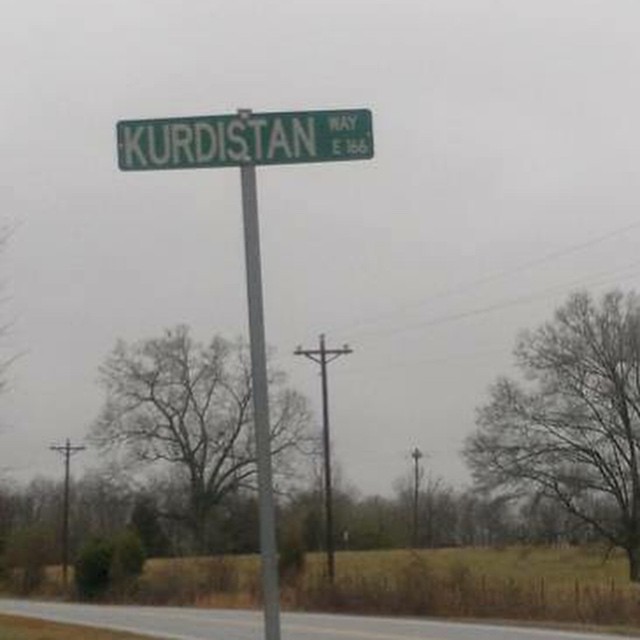The image captures a first-person perspective of a street scene centered around a street sign mounted on a very skinny, tall, gray pole. The rectangular sign, positioned horizontally and featuring a green background with white capital letters, reads "KURDISTAN WAY E 166." In the background, an asphalt roadway runs through the right side of the image, bordered by a small farm fence. The scene also includes power poles with wires strung across them, visible behind the street sign. The surrounding field appears predominantly green and brown, indicative of fall or winter, with most of the grass dying. The landscape features a tree without leaves on the left and another on the right side of the image, along with various shrubbery. Further back, additional trees frame the background, enhancing the rural ambiance.